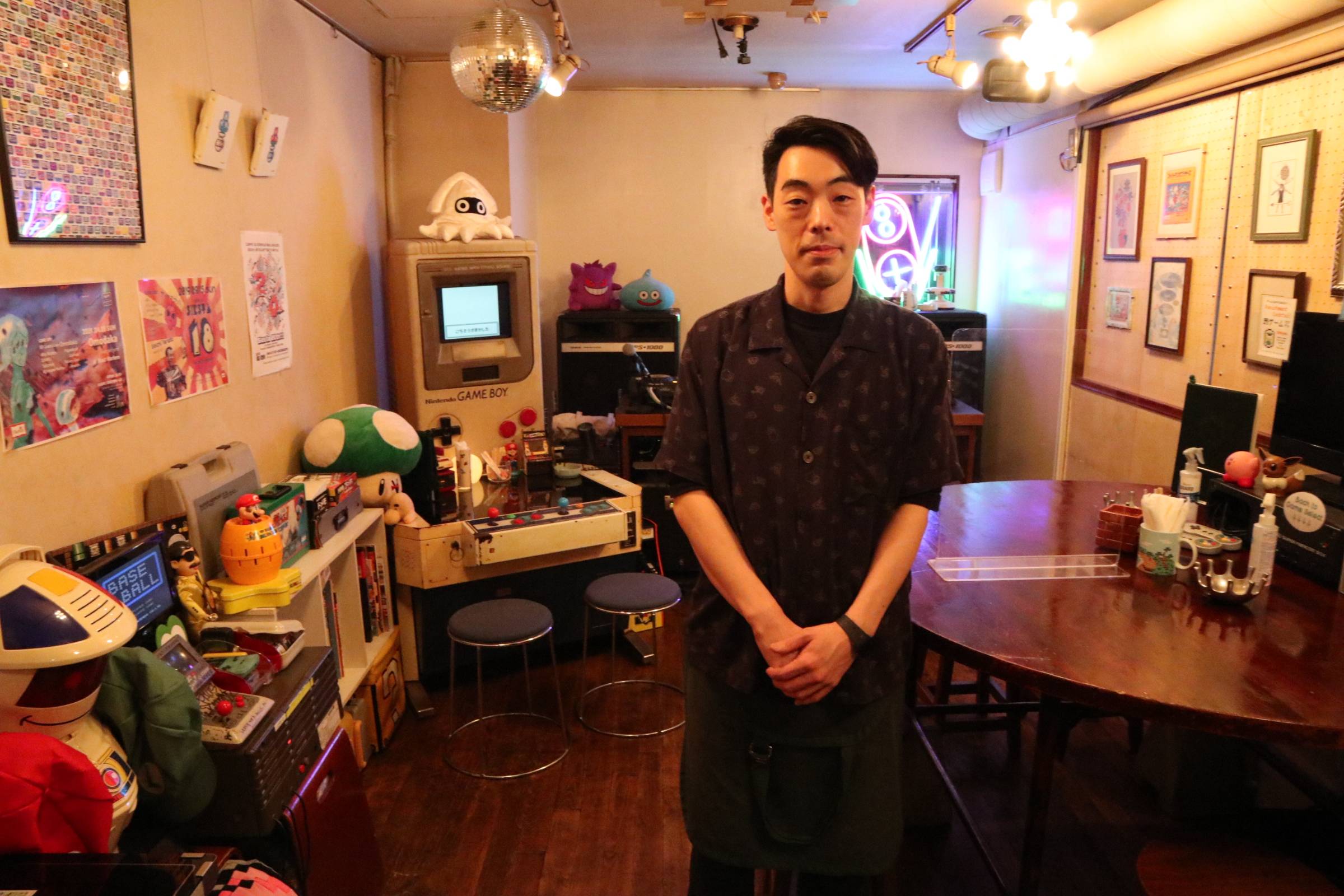In a warmly lit room filled with nostalgic memorabilia, a slim Asian man stands with his arms neatly crossed in front of him. He has dark, thick, medium-length hair styled with bangs and is wearing a black, short-sleeved, button-down shirt, along with a black watch. Consciously posing for the camera, he slightly smiles, looking directly into the lens.

Behind him is a kitchen table with two blue-cushioned chairs and a variety of items including a coffee mug, two spray bottles, and a computer monitor. To his right is a table housing a TV flanked by speakers, with two Super Nintendo controllers lying on it. The walls are adorned with numerous pictures and a collection of Nintendo or Mario-related paraphernalia, showcasing his evident passion for gaming.

Notably, in the left corner of the room stands a distinctly large Game Boy-style arcade machine, resembling an oversized handheld console fitted with joysticks and accompanied by stools. This space also features plush toys shaped like popular video game characters, including a mushroom character from Mario, a Pokéball, and a slime from the Dragon Quest series. Adding a final touch to this eclectic atmosphere is a disco ball hanging from the ceiling, emphasizing the blend of nostalgia and modern gaming culture that fills the room.